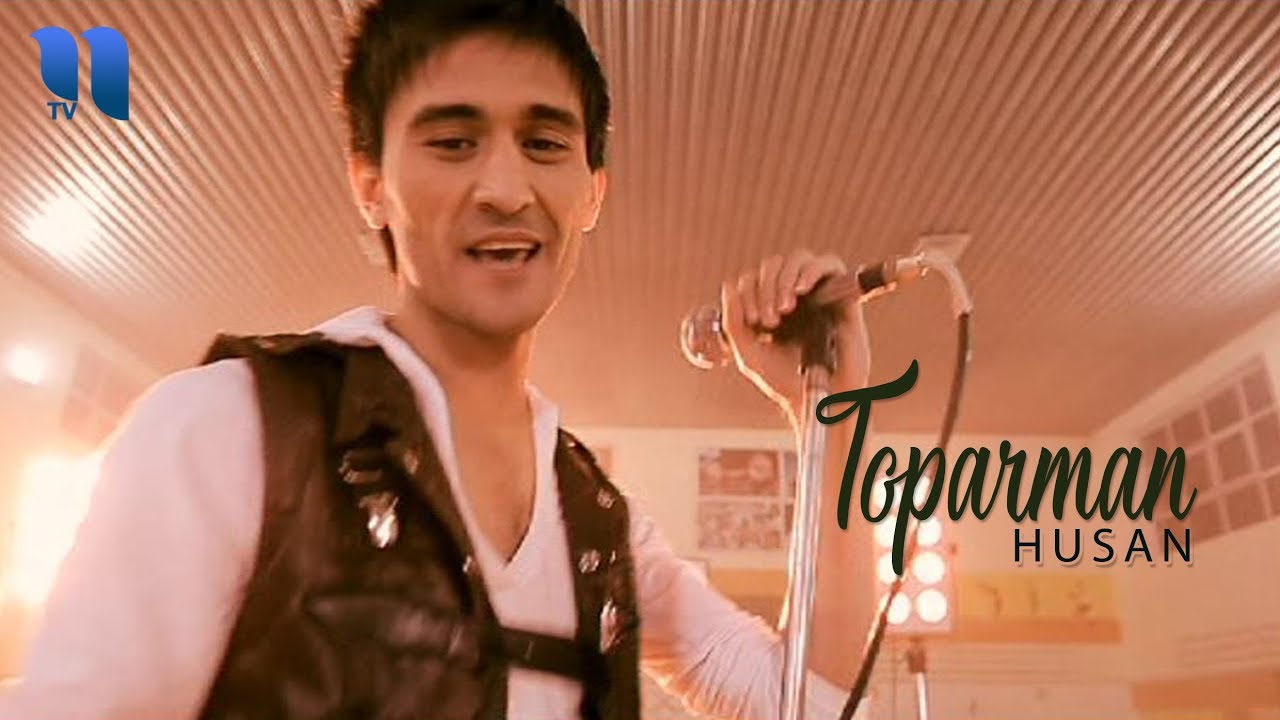The image depicts a man in an indoor setting, holding a standing microphone with his left hand, seemingly singing while gazing downward. He sports a short haircut and is dressed in a brown leather buckled vest over a white long-sleeve t-shirt. The room features a light brown, ribbed-patterned ceiling, with white walls adorned with many pictures. The background has a pinkish hue. In the upper left corner, there are two blue lines, potentially resembling a quotation mark or the number "11," with "TV" written beneath them, hinting at a possible television broadcast. To the left of the man, two lines of black text read "Thorpe Hermann Husen," with "Thorpe Hermann" in cursive and "HUSEN" capitalized.